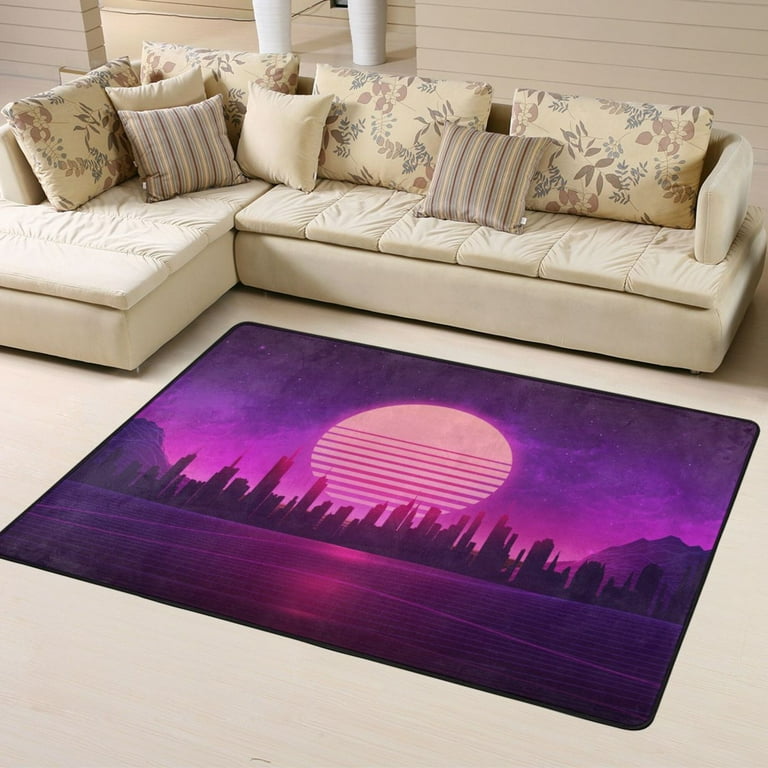A cozy living room scene features a long, beige, L-shaped sectional sofa adorned with an assortment of cushions. The cushions vary in size, with large horizontally rectangular ones displaying yellow leaf-like patterns, and smaller square ones in beige or adorned with brown, light brown, and yellow vertical stripes. Behind the sofa, a brown wall with white columns contrasts with the light hardwood floor beneath. Centered prominently in the room is a vibrant purple rug that captures immediate attention. This rug showcases an intricate design of a city skyline silhouetted against a moonlit backdrop, where the moon, in bright yellow hues, casts its glow over what appears to be water reflecting the cityscape. The entire carpet scene is rendered in striking purples, with pink and fuchsia accents, enhancing the imaginative and artistic ambiance of the living space.